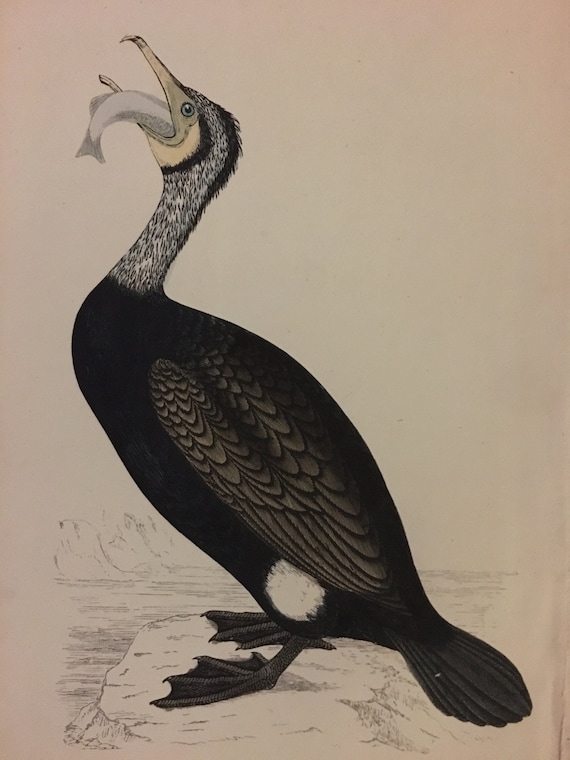This is an intricate black-and-white drawing of a water bird, likely a duck, captured in the act of swallowing a fish. The bird is positioned in profile facing right, with a medium-long neck adorned with white and yellow specks extending down to its black feathered body. The bird's face is a light tan or yellowish-beige, displaying an open beak that holds a small grey fish, which is partly visible with about 40% of its body inside the bird's mouth. The scene is set against a muted pinkish-gray background that suggests an environment of water and possibly cliffs in the distance. The bird stands firmly on a rock or embankment with its large webbed feet, hinting at a cold, aquatic habitat. The detailed portrayal captures the bird's intense moment of attempting to swallow its prey amidst a serene backdrop.